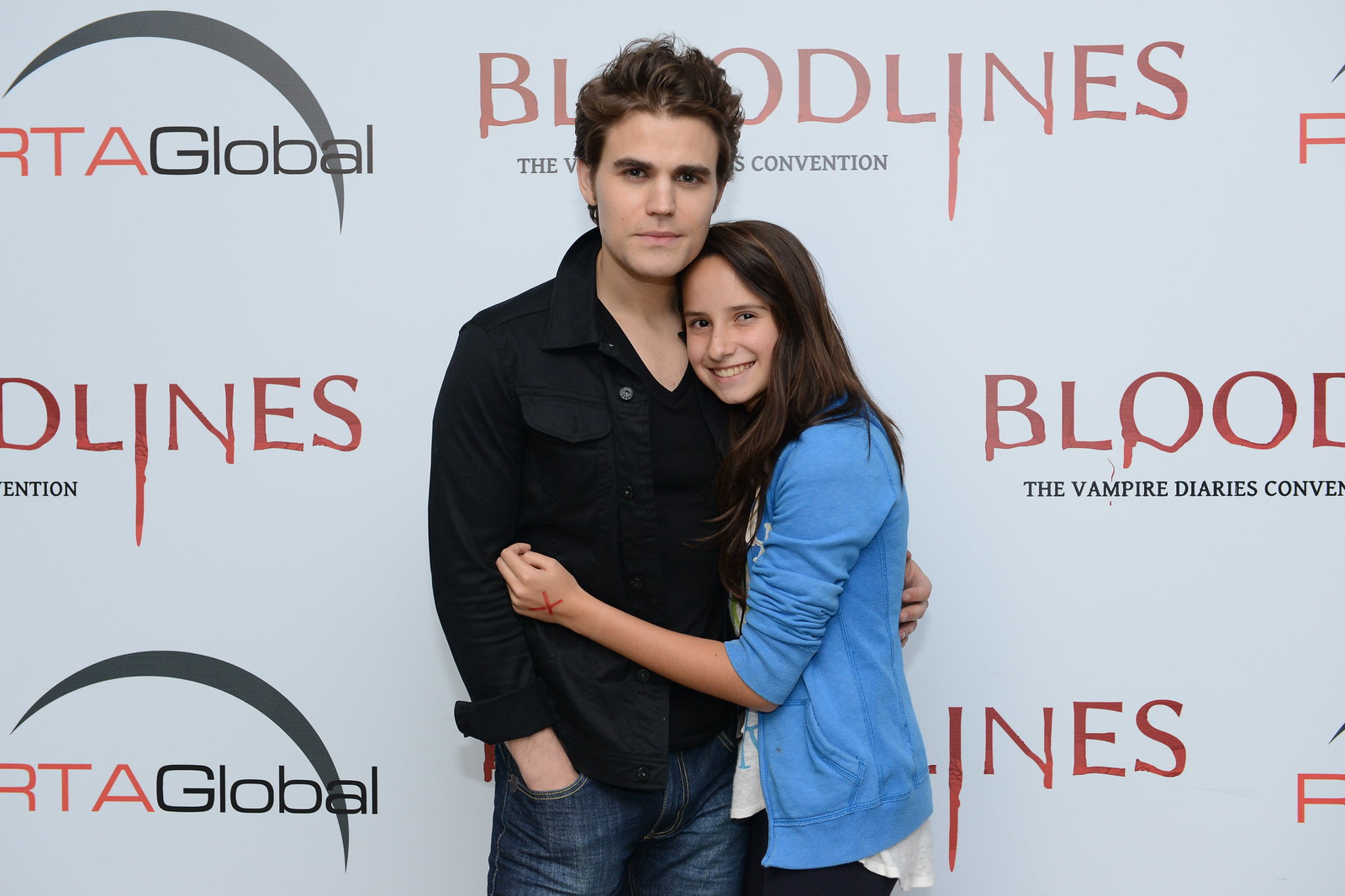The image depicts a young man and a young woman posing together in front of a backdrop at a convention. The backdrop prominently features the repeated text "Bloodlines The Vampire Diaries Convention" and "RTA Global." The young man, who appears to be in his 20s, has short, wavy dark hair and dark eyes. He is dressed in a black v-neck t-shirt layered under a black button-down collared shirt, paired with blue jeans. He exudes a casual yet attentive presence, with one hand in his pocket and the other hand wrapped around the young woman.

The young woman, identified by her long dark brown hair that cascades below her shoulders, is wearing a light blue hoodie over a white shirt and black pants. She is smiling and has her arm draped across the young man. Notably, she has a red X marked on her hand, suggesting that she might be a fan who paid to take a photo with the actor at the convention. The duo's pose and the setting give off a friendly, approachable vibe, indicative of the typical photo op experience at fan conventions.